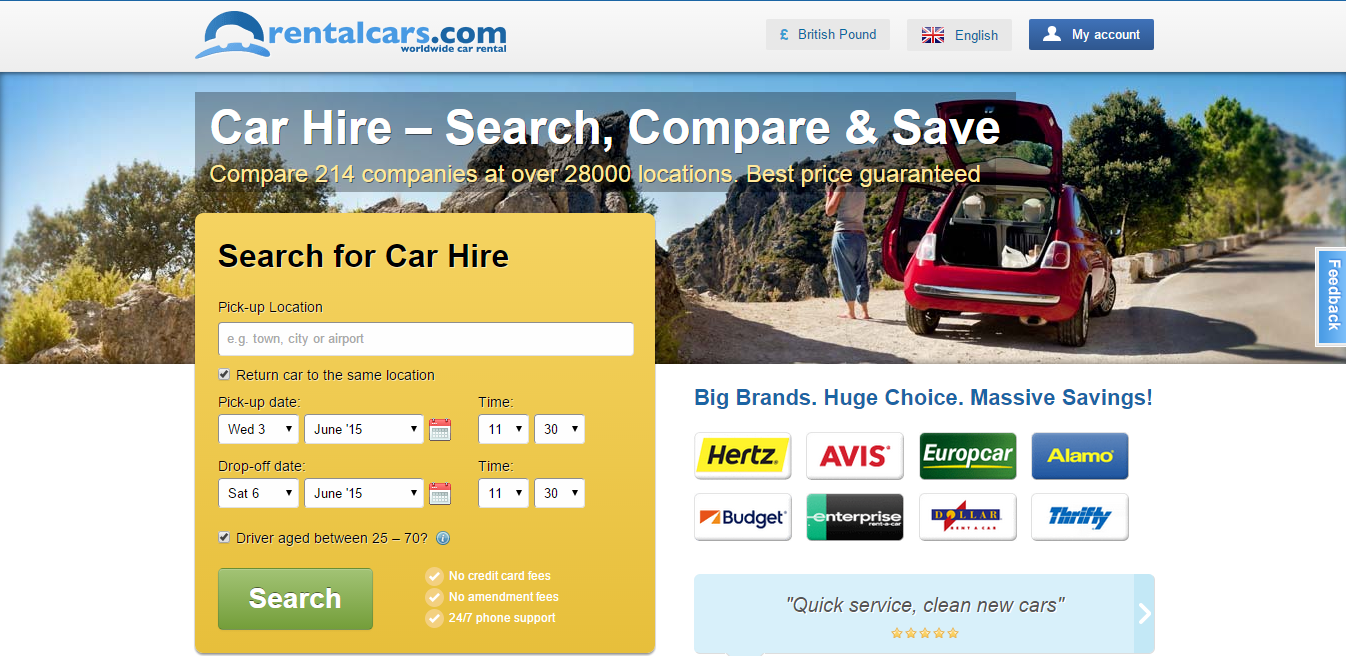The image features a visually structured advertisement for a car rental service. 

At the top, there is a white border with the text "rentalcar.com" in blue, followed by "Worldwide Car Rental." To the right, there is a representation of the British pound, including the pound symbol (£), labeled "British Pound." An English flag is also depicted next to the currency information.

Beneath the header, a dark blue rectangular box contains the text "My Account." Underneath this section, there's a prominent image of a burgundy car situated on the side of a road, with both the trunk and a door open. A woman is standing beside the car, seemingly engaged in a phone call.

Overlaying this image is a transparent box with the text "Car Hire - Search, Compare, and Save. Compare 214 companies at over 28,000 locations. Best Price Guaranteed."

Below this, there is an orange box prompting users to "Search for Car Hire." It includes a text box labeled "Pick-Up Location" which accepts input such as town, city, or airport. A checked box indicates the option to "Return Car to the Same Location." Additionally, there are drop-down menus provided to select the day, date, and month for the car hire.